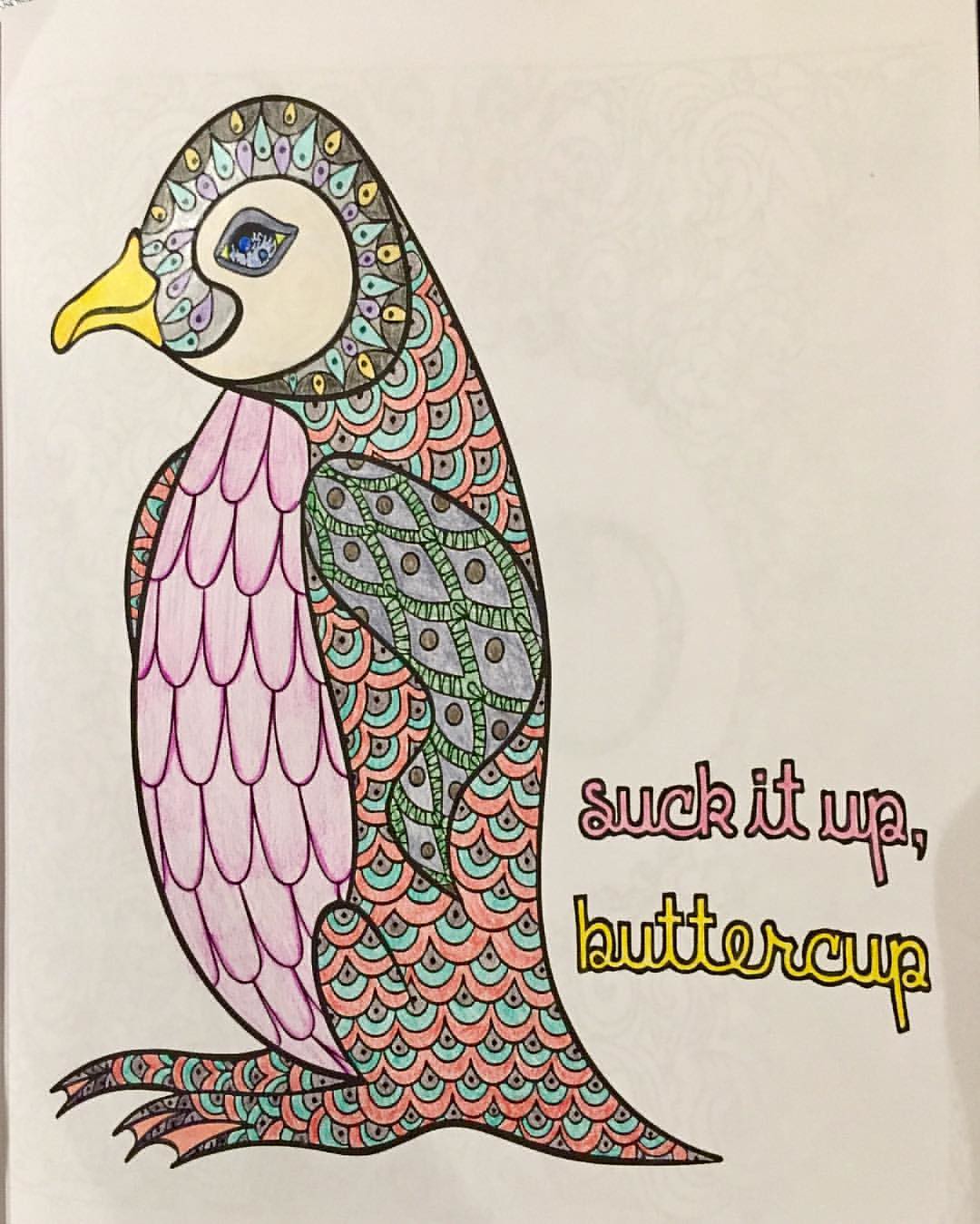This vibrant illustration showcases an unusually colorful penguin adorned with various eye-catching patterns instead of the traditional black and white. The penguin features a geometric, circular pattern on its back in hues of orange, green, and purple. The chest is painted a striking pink, and the wings display a mix of purple, green, and gray with dark dots and green stripes. The belly, resembling scales, is a purplish shade. The eye is an intricate combination of blue, black, and yellow. The rest of the body is decorated with scale-like patterns in red, green, and brown. The beak remains the only conventional part, painted a familiar yellow. To the right of the penguin, in a mix of pink and yellow cursive lettering, is the playful text: "Suck it up buttercup." The artwork has a coloring book style, suggesting it could be an interactive piece. The penguin stands on webbed feet, completing this whimsical piece.